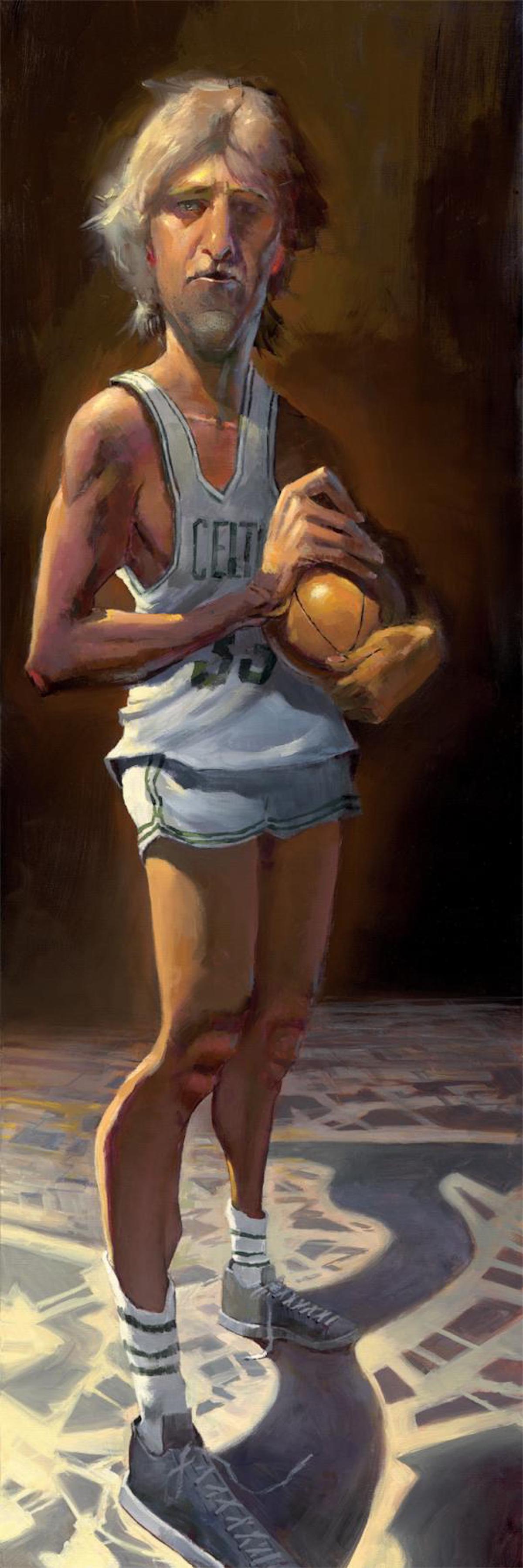The image is a vertically rectangular painting without a border, featuring a caricature of a Caucasian male basketball player, likely Larry Bird. The player is wearing a white Celtics tank top with the number 33, white shorts, white tube socks with striped bands, and gray shoes. He has long, shaggy blond hair and a clean-shaven face with a noticeable five o'clock shadow. The player holds an orange basketball that appears tiny due to his unusually large hands and elongated fingers. His calves are disproportionately big compared to his thighs, and his right leg has an odd, broken appearance around the knee due to skewed perspective. The background consists of a plain brown wall and a gray decorative floor with white lines and shapes.